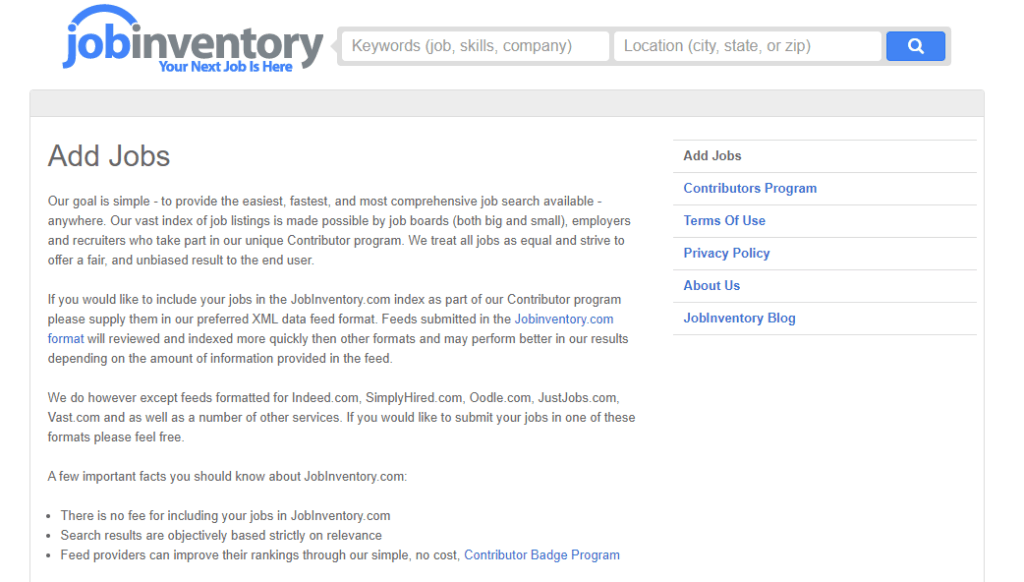This image is a detailed screenshot of a web page from the company "Job Inventory." The page features a clean, white background with various interactive elements for job searching. At the top left of the page is the company’s title, "Job Inventory," displayed in a distinctive lowercase format: "job" in bold blue font and "inventory" in gray. Above the word "job," there is a subtle semicircle that arcs over the text, resembling a rainbow.

Directly beneath the company’s name, a tagline in blue text reads, "your next job is here." Below this tagline, there is an intuitive search bar for users to input "Keywords, Job Skills, Company" in gray text. Adjacent to this, another search field prompts for the "City, State, or Zip" in parentheses. These search boxes are followed by a blue search button adorned with a magnifying glass icon.

The middle section of the page contains informative text around the purpose of the website: "Add Jobs. Our goal is simple, to provide the easiest, fastest, and most comprehensive job search available." The section ends with key bullet points emphasizing that "there is no fee for including your jobs," highlighting the site's beneficial features.

On the right side of the page, there is a vertical menu comprising five buttons. The top button, labeled "Add Jobs," is black, signifying a primary action. The subsequent blue buttons include "Contributors Program," "Terms of Use," "Privacy Policy," "About Us," and "Job Inventory Blog."

Overall, the layout is user-centered, offering easy navigation and clear instructions, enhancing the job search experience.